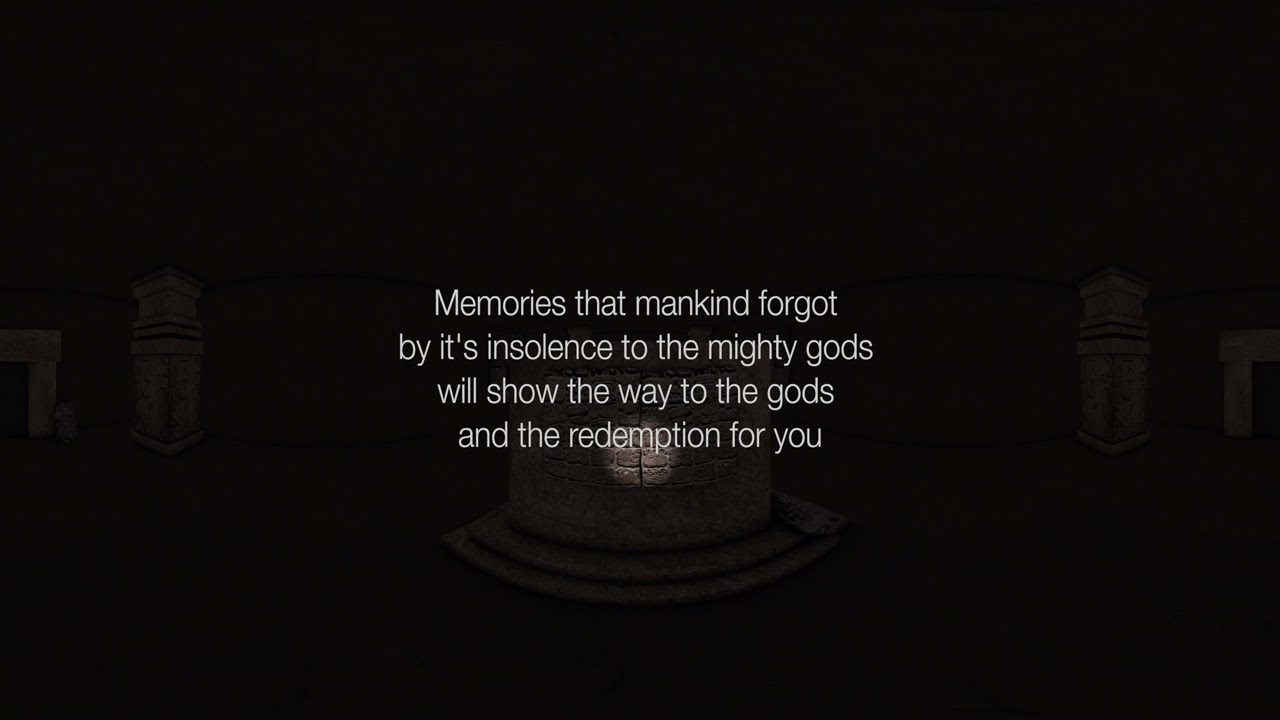The image depicts a very dark scene with a black 16:9 rectangle as the background. Faintly visible through a monochromatic overlay, approximately at 10% opacity, are indistinct stone pillars or monuments, suggesting a shadowy, mysterious environment. In the center of the image, a paragraph of white, sans-serif text is prominently displayed. The text reads: "Memories that mankind forgot by its insolence to the mighty gods will show the way to the gods and the redemption for you," with a minor grammatical error where "its" should not include an apostrophe. Behind the text and centrally located, there is an illuminated circle on a stone surface, possibly indicating an altar with steps leading up to it, evoking the sense of a sacred or ancient setting. The atmosphere is further emphasized by a spotlight effect that barely outlines the features in the dim environment.